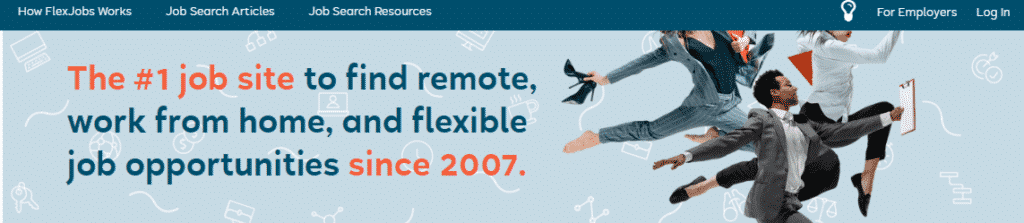This webpage snapshot from FlexJobs features a dark blue banner at the top with a thin ribbon that displays navigational links in white text: "How FlexJobs Works," "Job Search Articles," and "Job Search Resources." To the far right of the ribbon is a light bulb icon, followed by links for "For Employers" and "Log In."

The section below this ribbon has a light blue background adorned with simple, white icons such as a desktop computer and squiggly lines. Dominating the scene are three joyful professionals leaping into the air in business attire. One woman at the back, dressed in a gray pinstripe suit, joyfully holds her black high heels in one hand while leaping barefoot. A man in a gray suit clutches a clipboard, appearing to run exuberantly. Another woman, wearing black capris and a white blouse paired with black loafers, is captured mid-leap, exuberantly expressing her excitement.